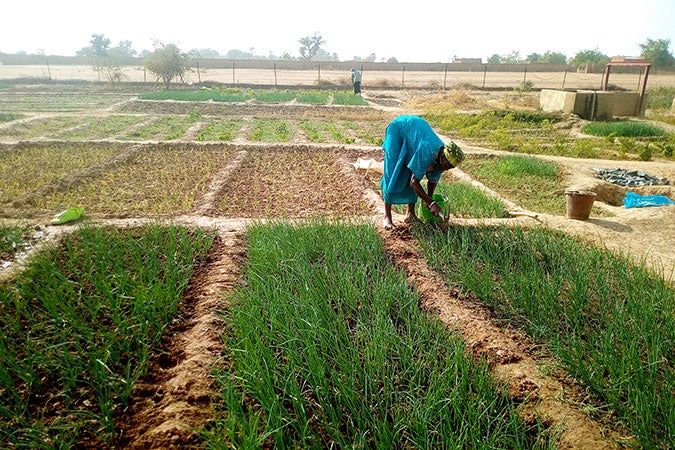In this photograph, an individual, possibly a tall and slender Black person, is depicted working diligently in an outdoor garden setting, possibly in Africa. They are wearing a yellow hat and a blue dress, and are currently bent over, tending to one of several enclosed garden beds which are at various stages of green growth. Specifically, they are working on a patch of thriving green grass, using a green watering can. Surrounding this patch are three other patches of grass and narrow dirt pathways. To the right, a brown bucket sits on the ground. The surrounding farmland appears dry and barren with multiple sections of enclosed gardens visible, along with a small structure and a large fence in the background. Farther off in the distance, there are a few trees under a bright white sky, suggesting a hot, sunny day.